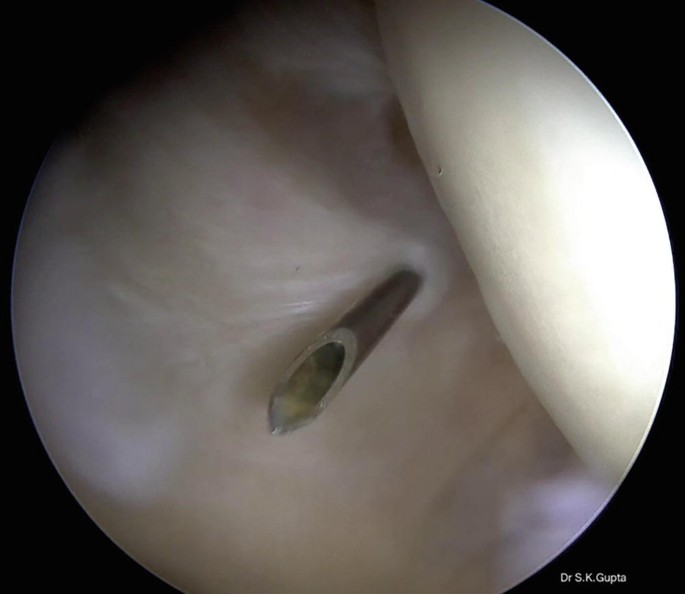The image features a large circular view set against a black square backdrop. Dominating the center is a silver needle that has pierced a white and pink tissue, likely part of a body, with what appears to be a slightly yellow liquid inside. The top and bottom of the circular view extend beyond the confines of the image, almost touching the left and right edges. The outer edges of the image are black, and in the bottom right corner, white text reads "Dr. S. K. Gupta." An additional flap with an even whiter color can be seen at the top right, partially obscuring the view. The overall impression is reminiscent of a medical camera capturing an internal procedure.